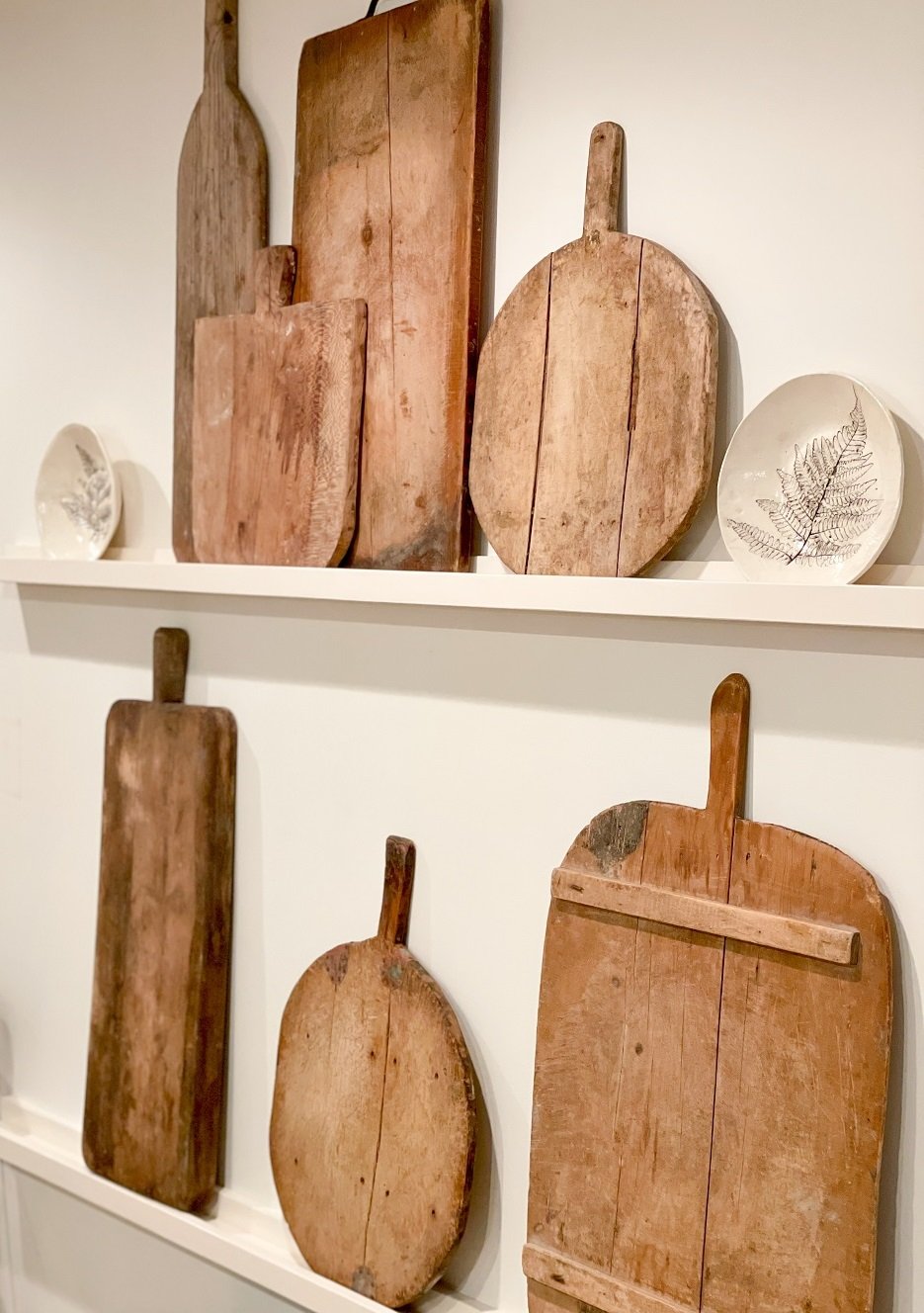The image depicts an assortment of old wooden cutting boards of varying shapes and sizes displayed on two thin shelves set against a tan background. On the top shelf, there are four different cutting boards, including a rectangular one and a round one, arranged between two small ceramic plates adorned with leaf prints in dark brown and silver hues. One smaller cutting board is positioned toward the left end of the right-hand plate, while another small, round cutting board is centrally placed on the bottom shelf. The cutting boards, which appear clean and well-maintained despite their age, suggest a historical significance, perhaps having been crafted many years ago.